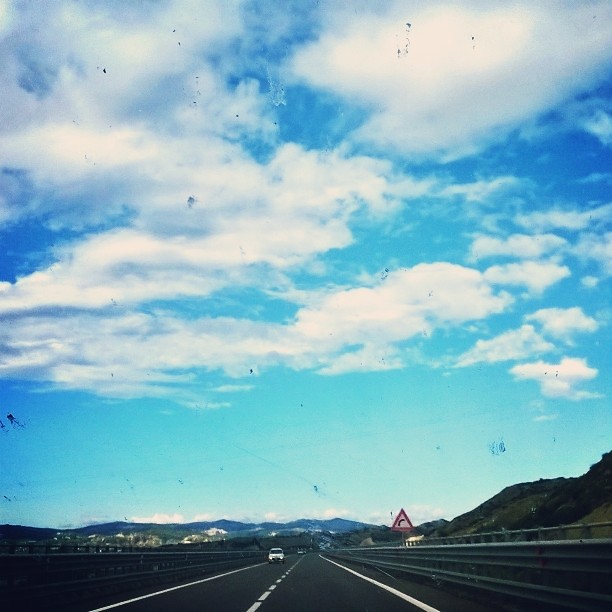This photograph captures a daytime scene on a two-lane highway nestled among the mountains. The expansive blue sky, occupying about 80% of the image, is dotted with prominent white clouds. The highway, bordered by solid white lines and flanked by steel guardrails, stretches into the distance, featuring a dotted white center line. 

Approaching the camera is a silver (or white) car with its headlights on, adding a sense of movement to the serene landscape. On the right side of the road, a triangular traffic sign with a yellow background and red border indicates a right turn with a curved arrow in the middle. Below this sign, a house with a gabled roof is visible, appearing to be directly under the sign from this perspective.

In the far distance, at the base of the mountain range, several houses or buildings can be seen, adding to the picturesque setting. The combination of the vivid blue sky, the majestic mountains, and the meandering highway create a strikingly detailed and atmospheric image.